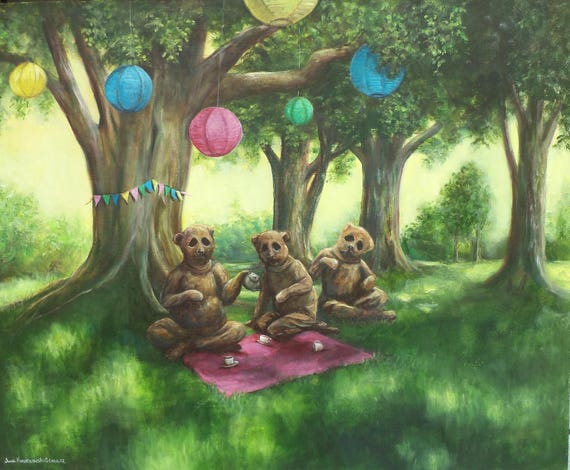The painting depicts a whimsical scene of three anthropomorphic bears having a festive picnic beneath a large, towering tree with a thick trunk. These bears appear more like people dressed in bear costumes, with the father bear on the left, the mother bear kneeling in the middle, and the younger bear seated on the right. The bears are arranged on a vibrant pink tablecloth, adorned with three coffee cups and a trio of lit candles. 

The backdrop is lush with tall trees, their green leaves stretching towards a yellowish sky that allows sunlight to sprinkle through and illuminate the verdant grass below. Draped across the main tree's trunk is a colorful banner featuring upside-down triangular flags in shades of blue, pink, yellow, and green. Similarly colored lanterns, resembling Asian-style round globes, hang from the tree branches above, adding a festive touch.

The serene picnic scene is captivating with its blend of natural elements and playful decorations, creating an enchanting forest setting. In the bottom corner of the image, there's a discrete signature in small, white font, adding a personal touch to this unique and detailed painting.